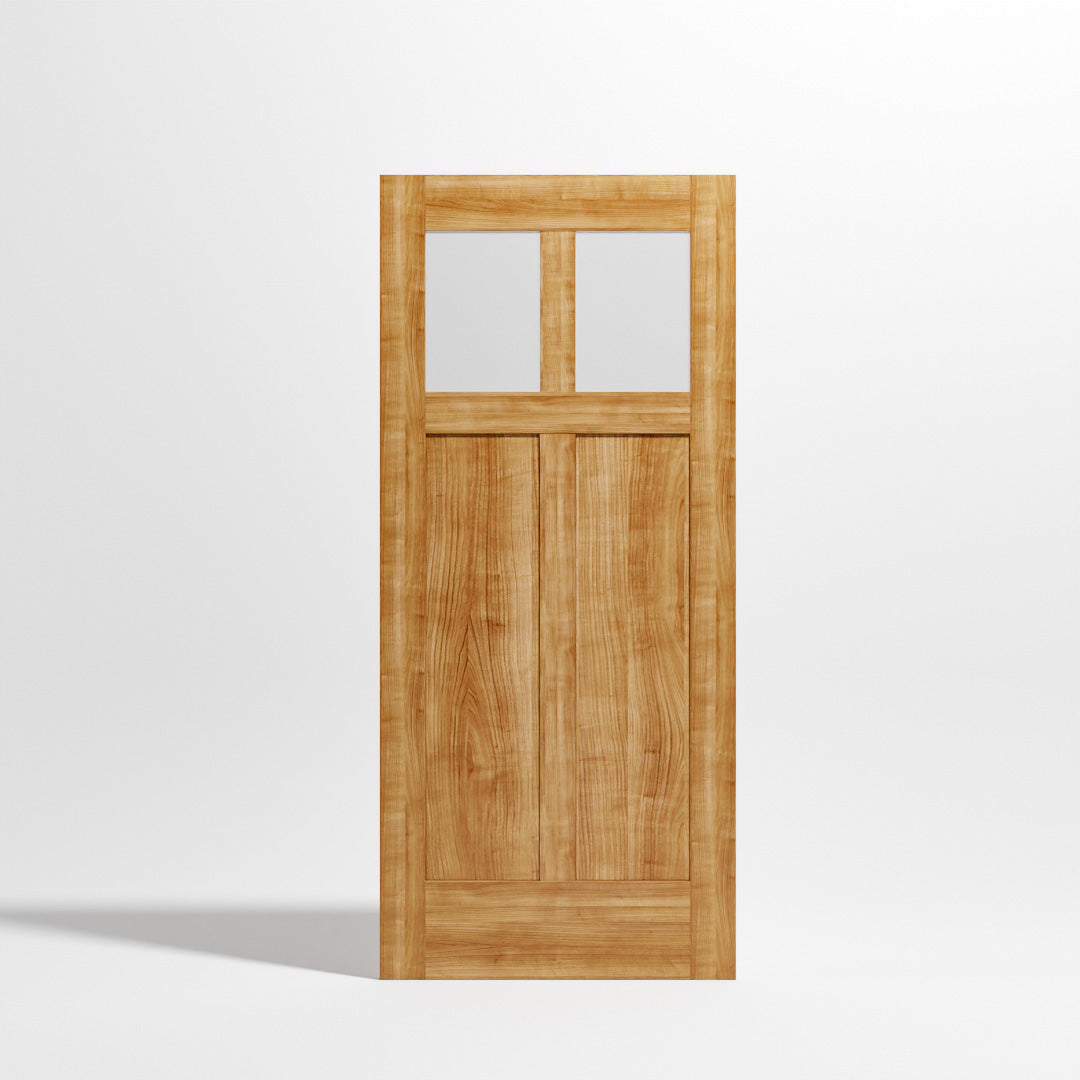The image showcases a freestanding, plain wooden door with a light brown hue, seemingly not connected to any structure. It's characterized by its unfinished, rustic look as if it hasn't been treated or varnished. The door is set against a plain, light grey background and casts a shadow to its left, indicative of lighting from the right. At the top portion of the door, there are two rectangular cutouts where windows would typically be, separated by a vertical wooden bar. This vertical bar continues downward and is intersected by a horizontal piece just below the cutouts, forming a cross shape in the upper quarter of the door. Below this section, the door is solid wood down to its base. Notably absent are any door handles, locks, or hinges, pointing to its depiction as possibly a digital rendering rather than a photograph. The door's minimalistic surroundings further emphasize its stark, standalone presence.